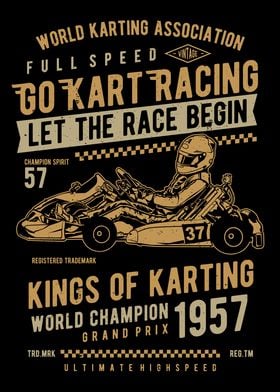This vintage go-karting poster from the World Karting Association features an eye-catching black background with dynamic yellow-gold text sprawled across it. Prominent phrases such as "World Karting Association," "Full Speed," "Go-Kart Racing," "Let the Race Begin," "Champion Spirit 57," "Kings of Karting," "World Champion," "Grand Prix 1957," and "Ultimate High Speed" create a thrilling atmosphere for enthusiasts. At the center, between "Let the Race Begin" and "Kings of Karting," a striking illustration of a go-kart racer in action is depicted. The racer, sitting in an open go-kart marked with the number 37, is clad in a coordinated orange suit complete with a helmet and gloves, adding to the poster's vintage appeal. The lack of speed lines or smoke suggests the kart might be stationary, underlining the timeless elegance of the design. Overall, this poster presents a nostalgic homage to the 1957 go-karting Grand Prix, capturing the ultimate high-speed champion spirit.